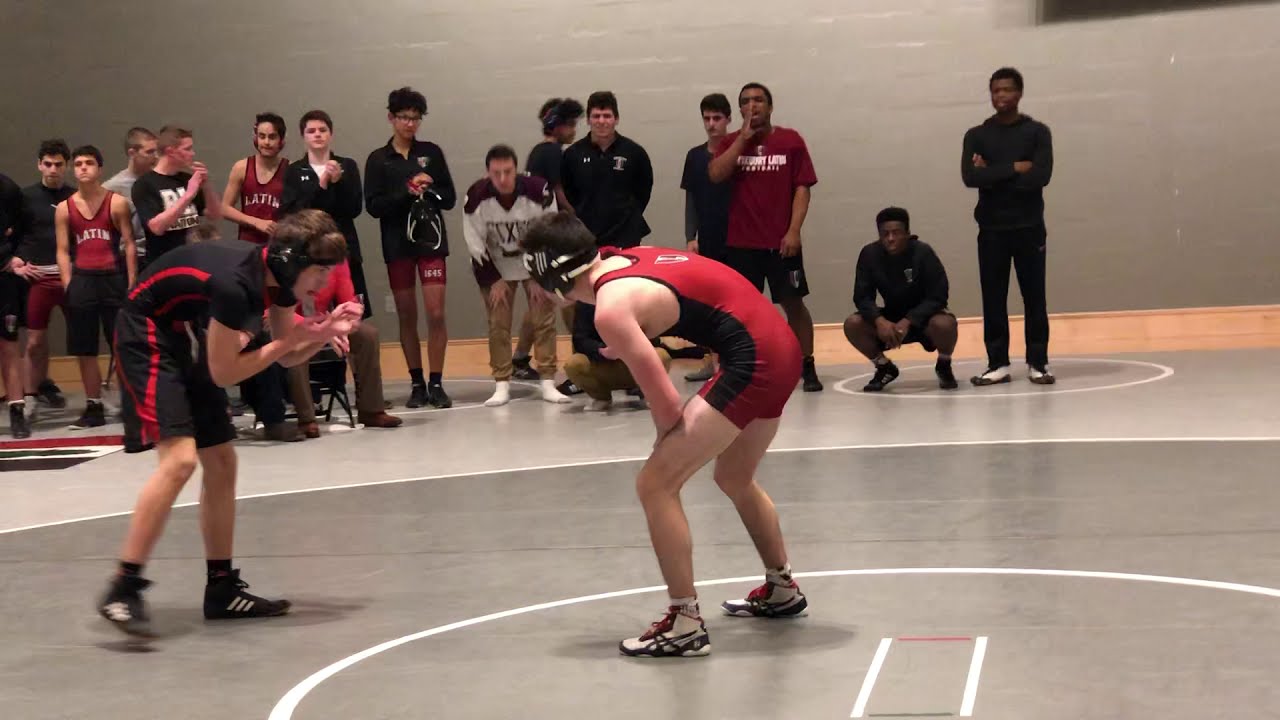This is a wide rectangular photograph capturing the intense moment before a wrestling match begins between two young adult males. The scene is set on a gray wrestling mat marked by two concentric white circles that curve from the left side towards the middle right of the image. Centered within the inner circle is a white wrestler clad in a red and black leotard, who is bent forward, facing the left. Opposite him, just outside the circle on the left, stands another white wrestler in a dark blue and red shorts and shirt combination, also bent forward in a ready stance. Both wrestlers are equipped with black headgear and display focused, intense expressions as they prepare to grapple. 

Surrounding the competitors is an animated crowd of young men, likely teammates and coaches, deeply engrossed in the match. Many of them wear red jerseys and sweat jackets, watching intently or cheering on the wrestlers. Most are standing, while one African-American gentleman at the end of the line is crouched down, and there is a man sitting in a chair, though his face isn’t visible. Their collective energy and anticipation add a palpable tension to the atmosphere.